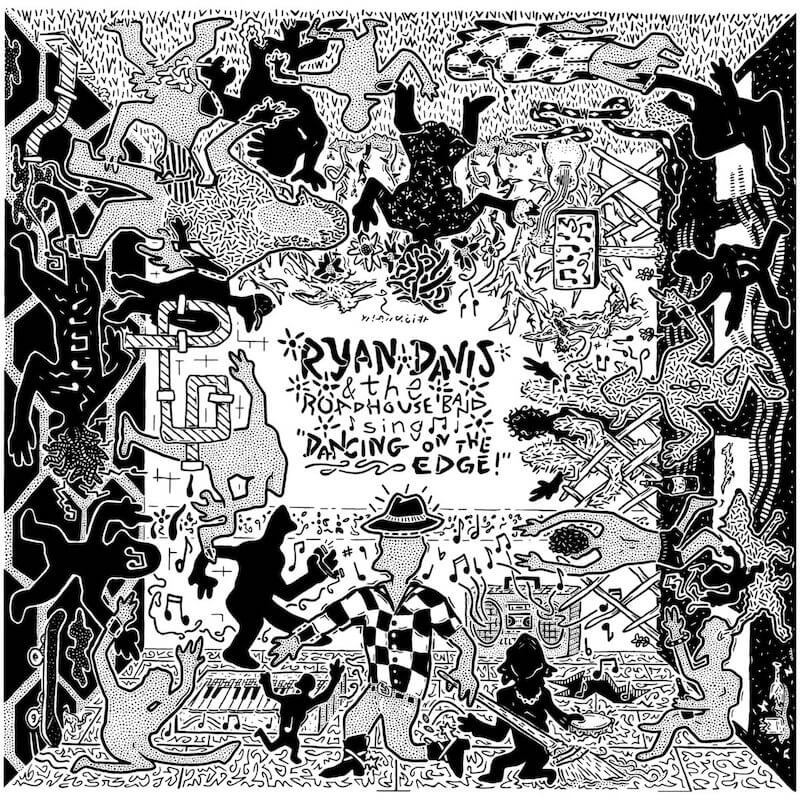This black and white stylized drawing serves as an advertisement for a concert by Rainn Davis and the Roadhouse Band, titled "Dance on the Edge." The busy illustration depicts a surreal, box-like room with people dancing on all four surfaces – the ceiling, floor, and walls. The focal point of the image is a man in a black and white check shirt standing upright in the middle of the floor, surrounded by musical notes and instruments, including a piano and a boom box. Scattered throughout the scene are shadowy figures, some partially dressed, and others are mere silhouettes. A notable detail includes a figure with snake-like hair hanging upside down. There are playful elements such as someone riding a dog and various abstract musical icons. Amidst this animated chaos, the central text announces the concert, emphasizing the lively and imaginative atmosphere of the event.